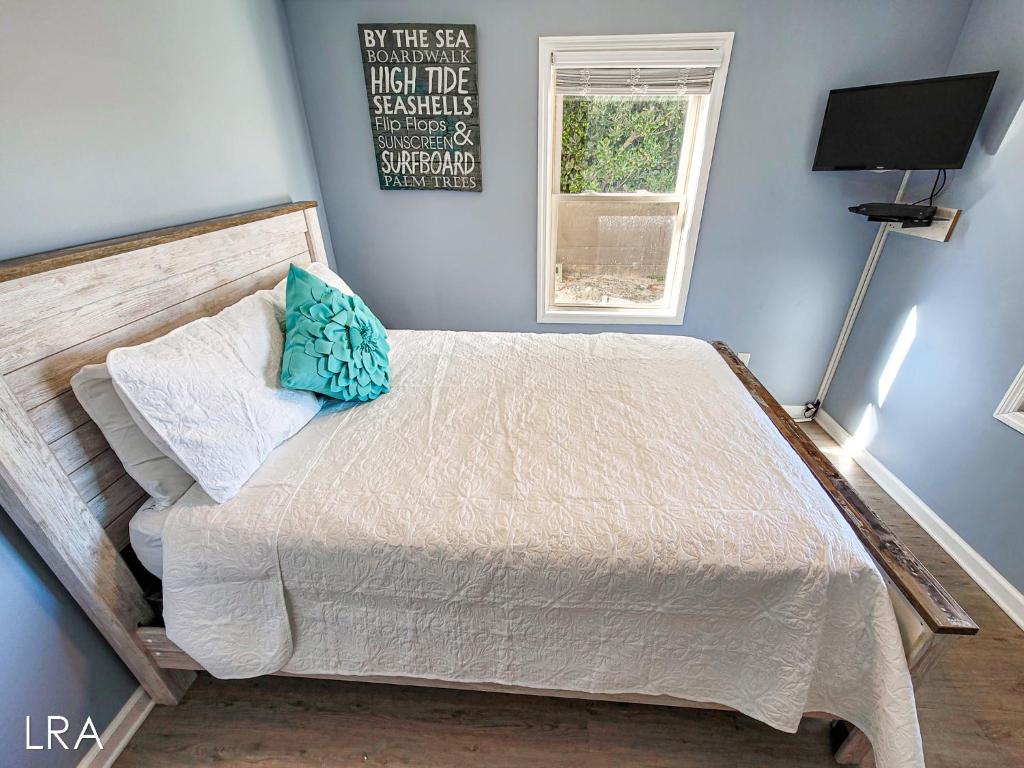This image depicts a cozy, small bedroom with light blue walls exuding a beachy, vacation vibe. Central to the room is a queen-sized bed, featuring a wooden headboard made of white planks. The bed is dressed in a cream-colored quilt with matching quilted pillow shams, accompanied by a teal pillow adorned with a flower design. On the right wall, a flat-screen TV is mounted, with a shelf and cable box nearby. A window, showing a glimpse of greenery outside, sits prominently on the back wall. To the window's left is a decorative plaque that reads, "By the Sea, Boardwalk, High Tide, Seashells, Flip Flops, Sunscreen, Surfboard, Palm Trees." The room also features rustic light wood flooring and white trim, and in the bottom left corner of the image, there's a watermark labeled "LRA."